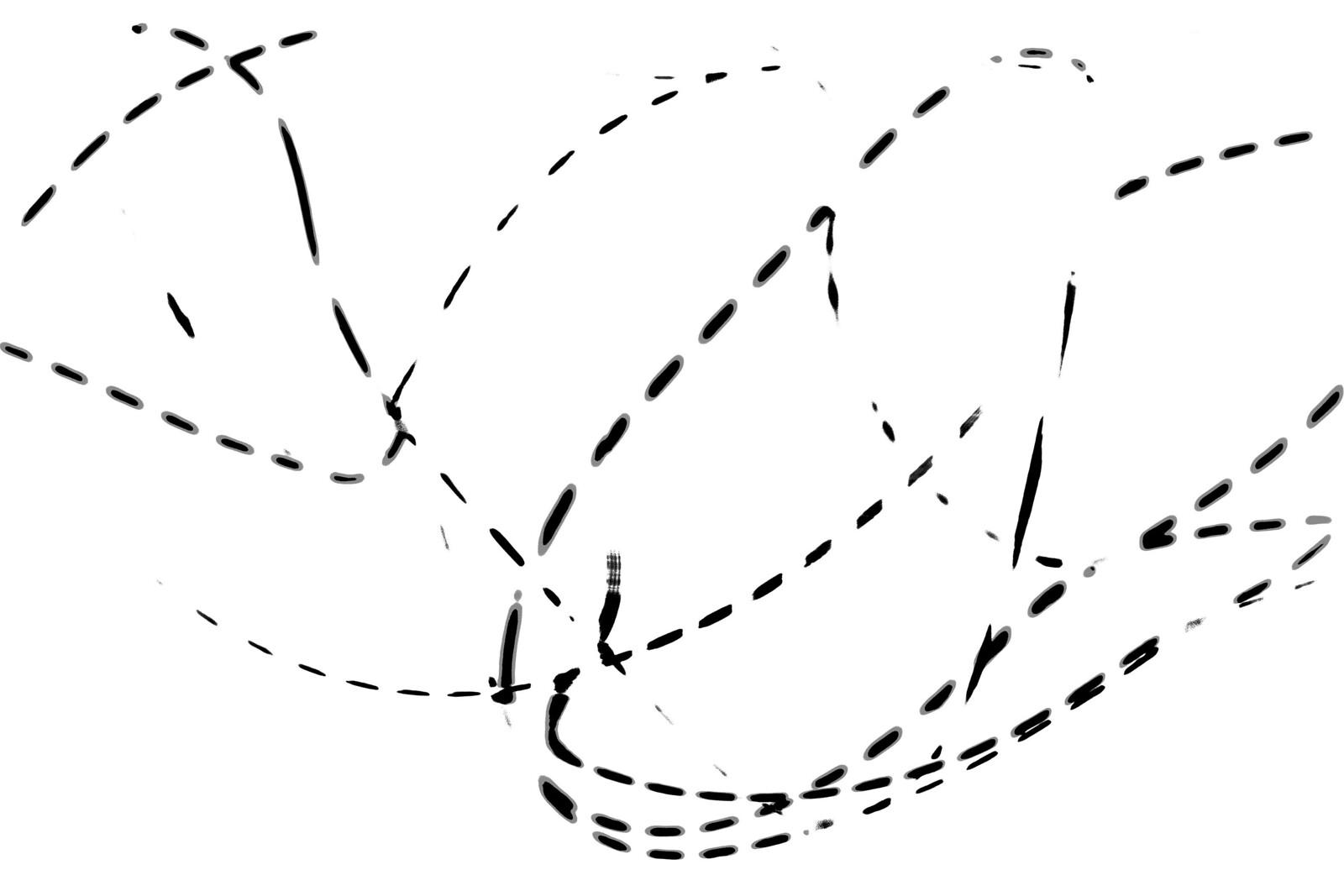The image features numerous irregular, dotted lines against a white background. These dots vary in length and spacing, creating an uneven and dynamic appearance. In the bottom right corner, the lines are particularly dense, forming intricate circular patterns. Moving upwards to the top right, the dotted lines converge into a near heart shape. From the center of this shape, a solitary line stretches downward almost reaching the bottom of the image. Adjacent to the top left of this heart shape, a prominent bold dotted line extends downward and slightly to the left, leading towards the bottom left corner. Additionally, in the top left section of the image, a rough triangular shape is distinguishable with a small dot placed centrally within it.